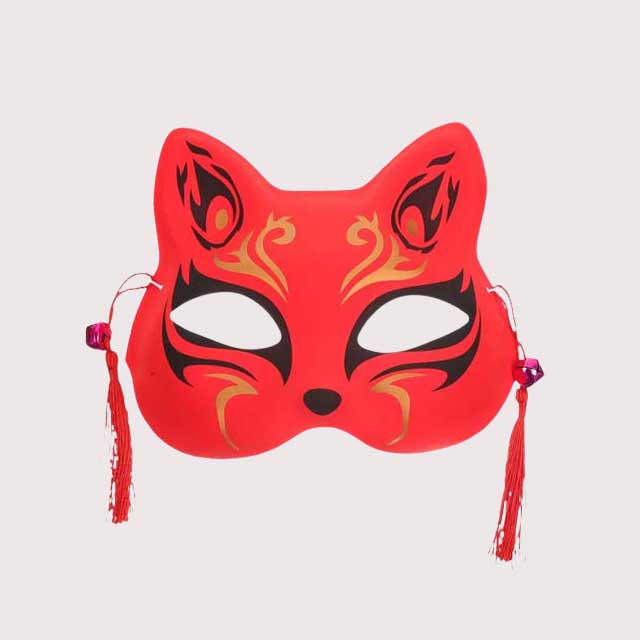This image depicts a highly detailed photograph of a red cat-shaped half-mask. The mask reveals the upper part of the face, such that the nose and mouth would remain visible when worn. It features almond-shaped eye cutouts surrounded by black designs that resemble flames. There is intricate black shading around the eyes and ears, with a black nose at the center of the mask.

The mask is decorated with gold details: gold is found above the eyes, mimicking eyebrows, and beneath the eyes, enhancing its ornate look. The ears also contain both black and specks of gold. Two red tassels with small pink bells or beads at the top are attached on either side, hanging down like whiskers. The mask is facade-sized, meaning it would cover the face perfectly.

The background of the image is white, making the mask’s vibrant colors stand out vividly. The mask’s elaborate design suggests it could be used for festivals, performances, or as a decorative wall piece.